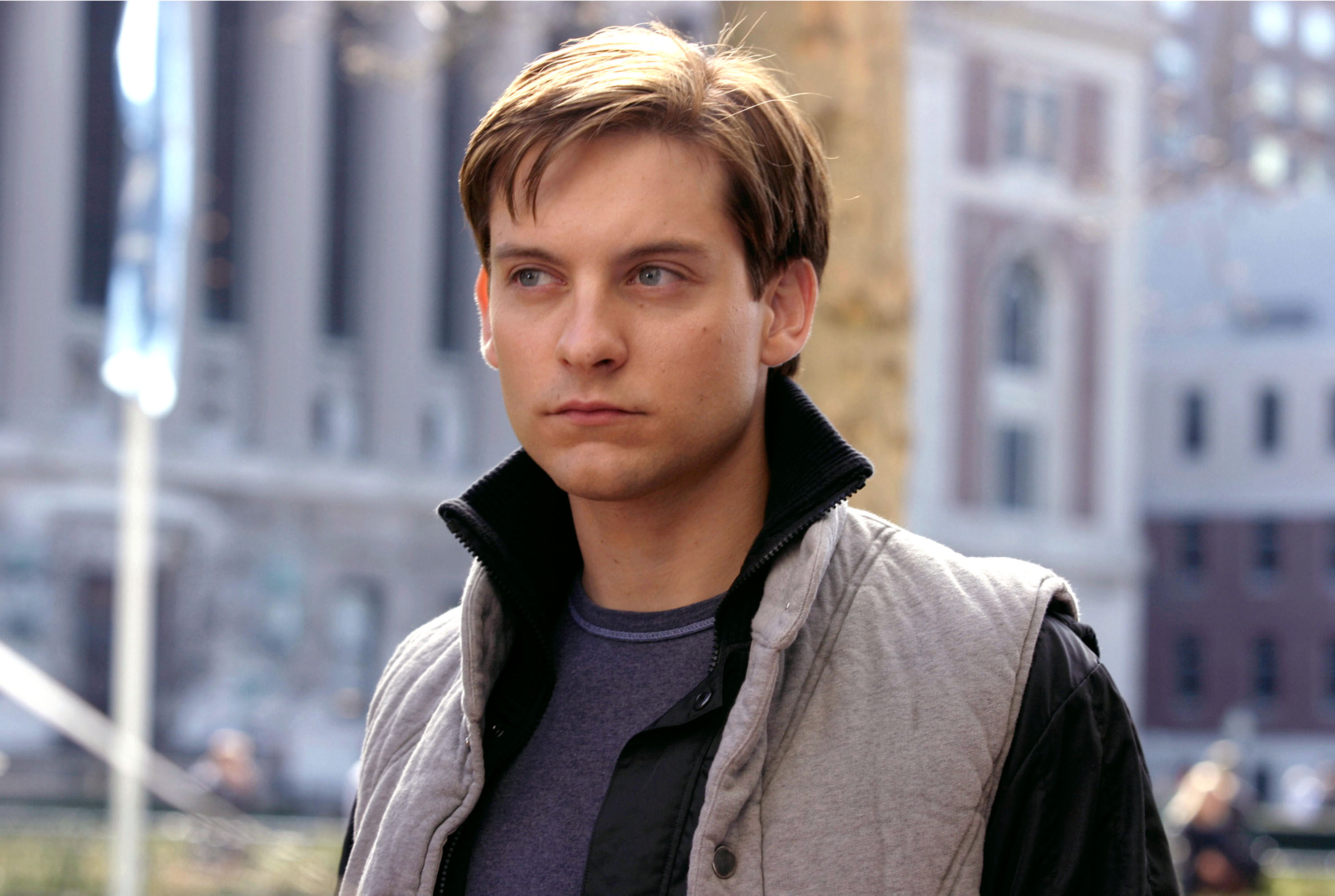The photograph features a young white male, likely in his late 20s to early 30s, with medium-length brown hair that is parted to the side and slightly covering his forehead. He has blue eyes, dark brown eyebrows, a smaller nose compared to his mouth, and fairly thin lips. He is dressed in a gray vest layered over a black jacket, and beneath that, a blue shirt with light blue piping at the neck. The man is looking introspectively into the distance. The urban background includes multiple buildings: a prominent large gray building with pillars, a white building with burgundy accents, and another structure with a white roof and dark brick exterior. Additionally, a blurred figure can be seen behind him.